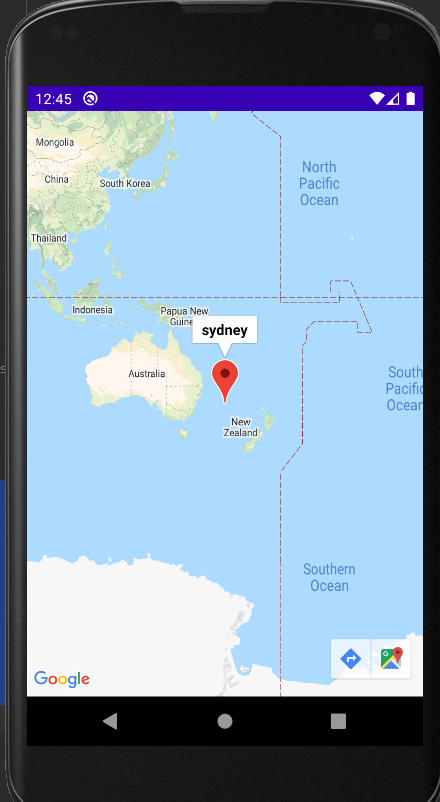The image displays a smartphone with a dark gray frame. The screen captures a detailed view, starting with a purple top border where the white font indicates the time as 12:45. It does not specify whether it's a.m. or p.m. The right side of the top border shows a fully charged battery icon, weak wireless connection signals, and a strong Wi-Fi connection signal.

Dominating the screen is a Google Maps view centered on Australia. The map also includes parts of Antarctica at the very bottom and a significant portion of Asia in the upper left corner, with countries such as China, Thailand, and South Korea specifically marked. The map labels the North Pacific Ocean, South Pacific Ocean, and Southern Ocean. A red location marker is prominently placed over Sydney, with the name "Sydney" written in lowercase letters within a white rectangle above the marker.

The bottom border of the screen is plain black, featuring a gray circle in the middle, a gray square on the right, and a gray rectangle pointing left. The bottom part of the smartphone is slightly cut off in the image.